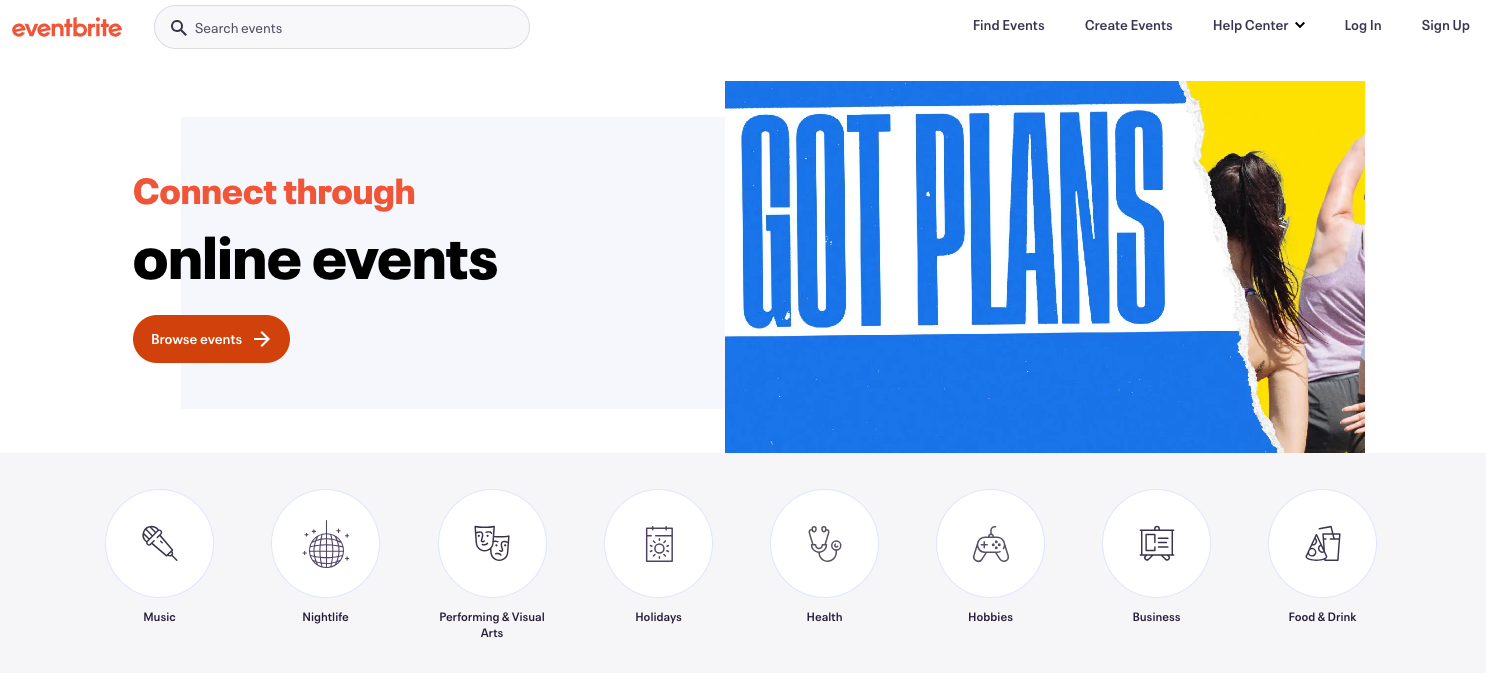#### Webpage Screenshot of Eventbrite:

In this screenshot of the Eventbrite homepage, the user interface is designed for easy navigation and user engagement. 

- **Top Left Corner:** The Eventbrite logo appears in lowercase letters, rendered in a vivid red color.
- **Top Center:** Adjacent to the logo is an oval-shaped search bar, facilitating user searches for events.
- **Top Right Corner:** A navigation menu lists five options in sequence: "Find Events," "Create Events," "Help Center," "Log In," and "Sign Up."
  
- **Main Section (Left Side):** Dominating the central area, text prominently reads "Connect Through Online Events," inviting users to explore various events.
  - Below this text is a significant red oval button labeled "Browse Events."

- **Main Section (Right Side):** A horizontally placed rectangular image adds visual interest. 
  - **Image Description:** 
    - The left half showcases a blue and white color gradient.
    - The right half transitions to a bright yellow.
    - Two partially visible individuals are situated on the right half; one has long, dark hair, and the other’s head is not visible, both depicted with light skin tones.

- **Bottom of the Page:** A horizontal toolbar runs across, featuring icons and links for various event categories:
  - Music
  - Nightlife
  - Performing and Visual Arts
  - Holidays
  - Health
  - Hobbies
  - Business
  - Food & Drink

This screenshot effectively captures the clean, user-friendly design of the Eventbrite homepage, emphasizing ease of access to event browsing and creation.